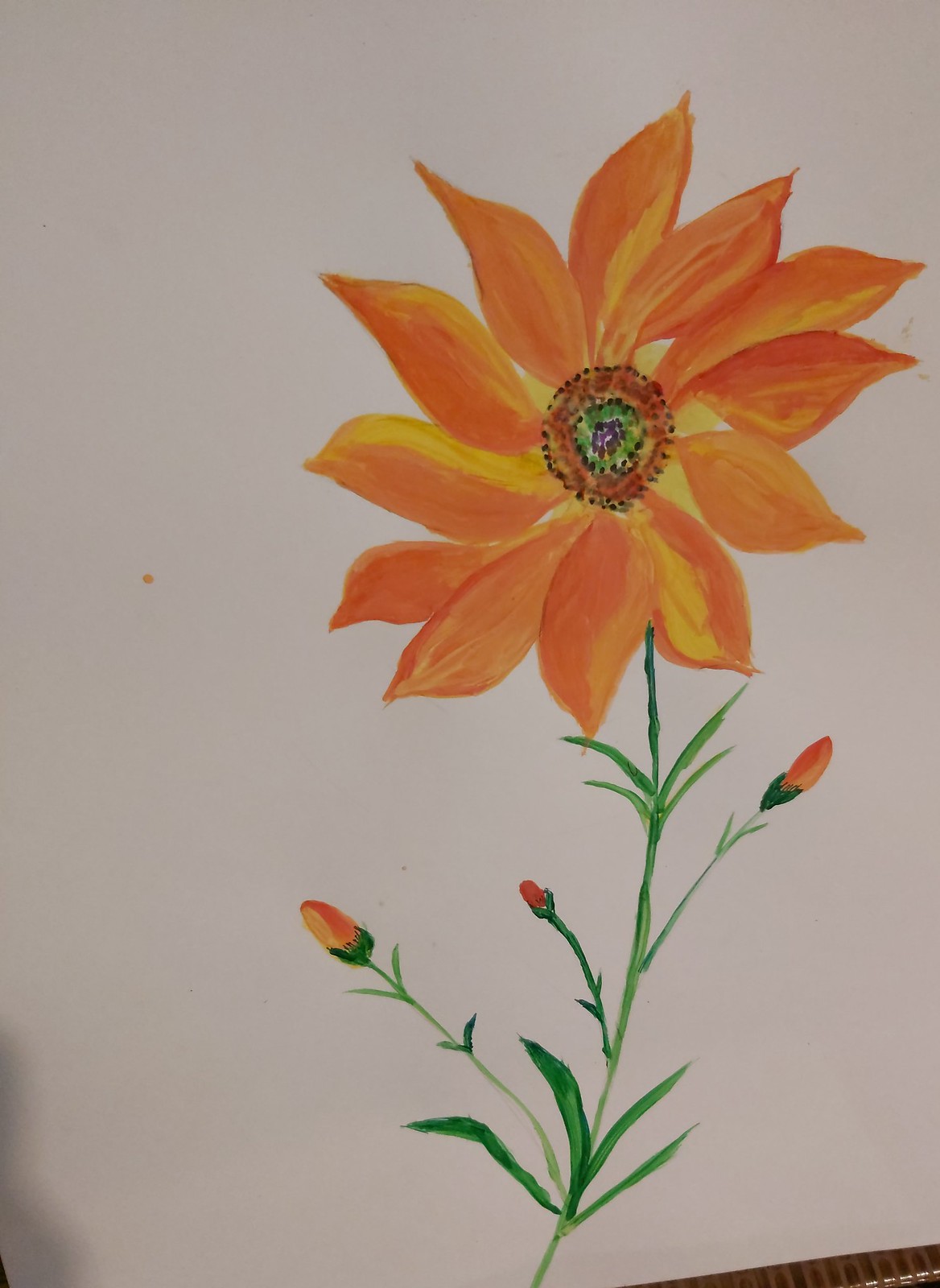A freshly made, colored pencil drawing of an orange flower stands out against a white piece of paper. The flower has large, overlapping petals totaling around 13, some with subtle yellow shading. At the center of the flower are concentric circles: starting with fine black dots, followed by a brown border, then more black dots, and finally a green ring leading to a core of tiny purple dots.

The stem, originating slightly right of center, is green and rises halfway up the image, branching out into smaller stems and leaves. On the lower part of the stem are pairs of green leaves extending to the left and right. Interspersed among these leaves are several slender stems, each bearing an undeveloped orange flower bulb. The arrangement of these unopened buds varies, with some extending left, others right, and a few pointing upward. A small, unintentional splash of orange is noticeable to the left of the main stem, adding an additional touch of color to the white background.